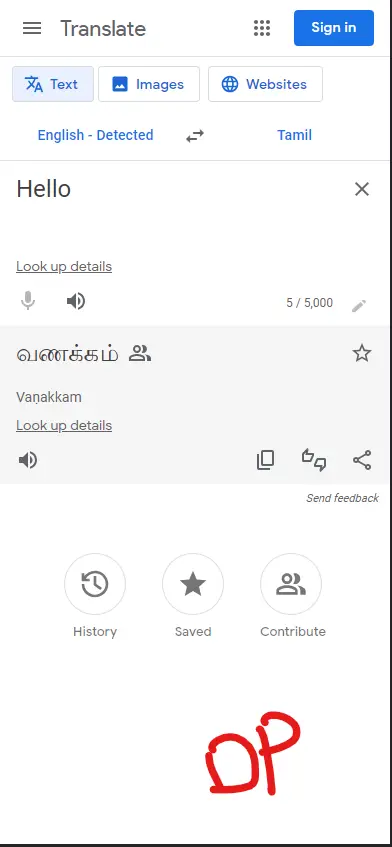This image is a detailed screenshot of the Google Translate interface. In the top-left corner, we see the familiar three horizontal bars that open a menu, with the text "Translate" displayed prominently next to them. Below is a dropdown menu icon allowing access to other Google applications and a blue "Sign In" button that indicates the user is currently not signed in.

Central to the image is the primary translation area, which is divided into two main sections. On the left, highlighted in input text, is the English word "Hello." This area is complemented by various interactive icons including "Speak" and "Play" buttons, which facilitate the audio pronunciation of the word. Additionally, it displays a character count, showing 5 out of a 5,000 character limit.

The right section of the main interface shows the translation into Tamil. Though the Tamil script cannot be read by the user, a transliteration "Vanakkam" is provided below, representing the phonetic pronunciation in English characters. This output box is equipped with several functional buttons: "Copy," "Paste," "Thumbs Up," "Thumbs Down," and "Share."

Further options for interaction include "History," "Save," and "Contribute" buttons below the translation box. The only other notable marking in this space is the hand-drawn red letters "OP" towards the bottom of the screen.

Lastly, the screenshot features a black border along the bottom and right sides, but not on the top or left. Overall, the image depicts a user (not signed into Google) utilizing Google Translate to convert the word "Hello" from English to Tamil.